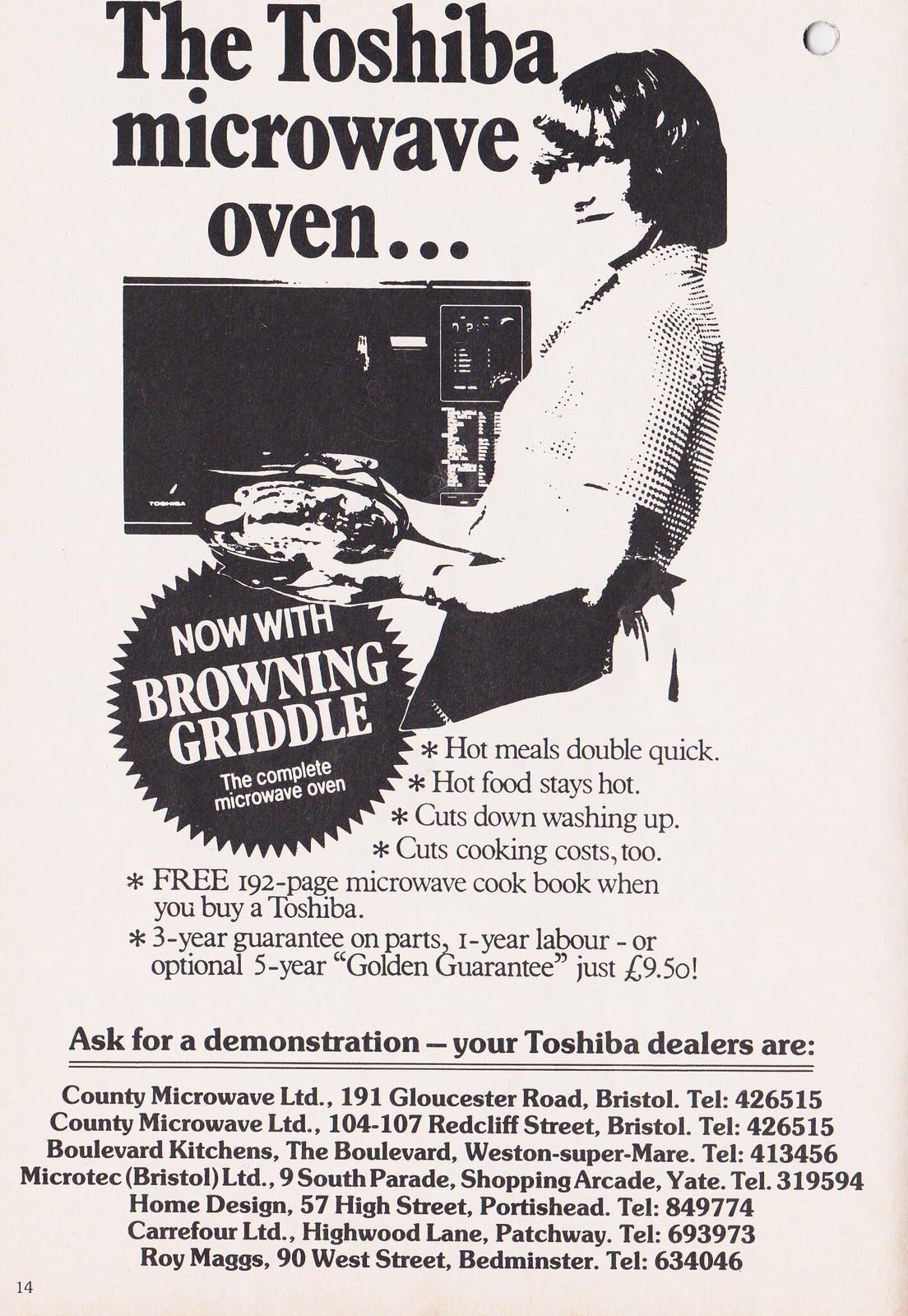This is a vintage advertisement for the Toshiba microwave oven, featuring a pale light blue-purple background. At the top, large text reads, "The Toshiba Microwave Oven..." Accompanied by an image, a smiling woman wearing an apron is pictured in front of a black microwave, holding a large platter of food ready to be placed inside. Beneath the image, the ad boasts about its latest feature, "Now with Browning Griddle, the Complete Microwave Oven." It lists several benefits including, "Hot meals double quick, hot food stays hot, cuts down washing up, cuts cooking costs too." Additional incentives are detailed: "Free 192-page microwave cookbook when you buy a Toshiba," and "Three-year guarantee on parts, one-year labor, or optional five-year golden guarantee for just £9.50." The ad concludes with a call to action, "Ask for a demonstration," followed by a list of Toshiba dealers. A small number "14" is present at the bottom left, indicating its placement in a magazine or catalog.